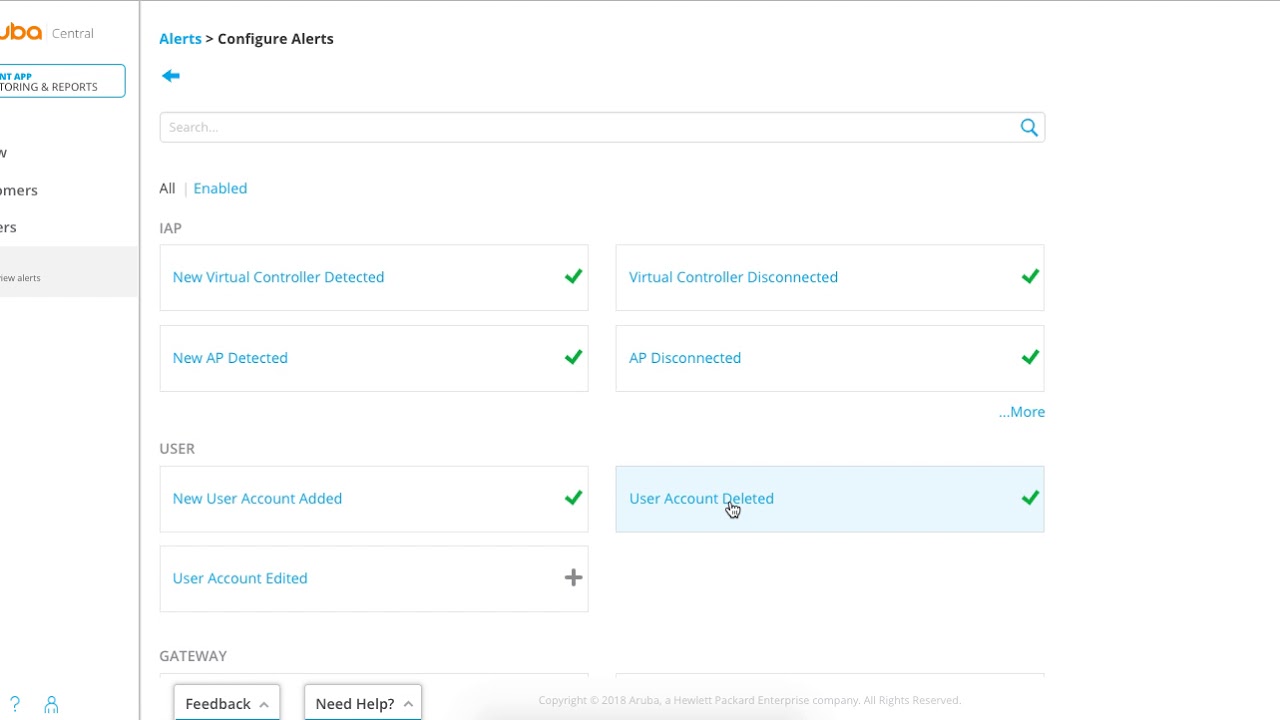A webpage layout dedicated to settings is visually described. On the left-hand side, partially visible orange text reads "UBA," with adjacent gray "central" text and a cyan-bordered rectangle containing "N-T-A-P-P" in cyan. Words "T-O-R-I-N-G and reports" in black follow, partially cut off. Below, segmented text reads "W," "M-E-R," and "O-F-S" on subsequent lines. A gray rectangle labeled "New Alerts" is also truncated.

The right-hand section features a prominent "Alerts" in cyan blue at the top, accompanied by a bold black arrow pointing right. Next, "Configure Alerts" appears in bold black. Below, a cyan blue arrow points left above a thin dark gray-bordered rectangle labeled "Search" in gray, capped with ellipses. A cyan magnifying glass icon occupies the far right of this rectangle.

Beneath, the word "All" in bold black precedes a gray line leading to a clickable "Enabled" in cyan blue. The section displays horizontally aligned rectangles, with one highlighted. The first, labeled "New Vertical Controller Detected" (marked with a green checkmark), features "I-A-P" in all caps and cyan blue text. Adjacent texts include “Virtual Controller Disconnected” and “New A-P Detected,” each with a green checkmark. Another highlighted item, "A-P Disconnected," follows.

Under the "User" heading in black, new rectangles appear: "New User Account Added" and "User Account Deleted," with the latter highlighted in light blue. A gray hand-shaped cursor hovers over it. The list continues with "User Account Edited" featuring a gray plus sign rather than a checkmark.

At the bottom left, the word "Gateway" precedes a horizontal gray line, followed by two buttons labeled "Feedback" and "Need Help," each marked with an up arrow.